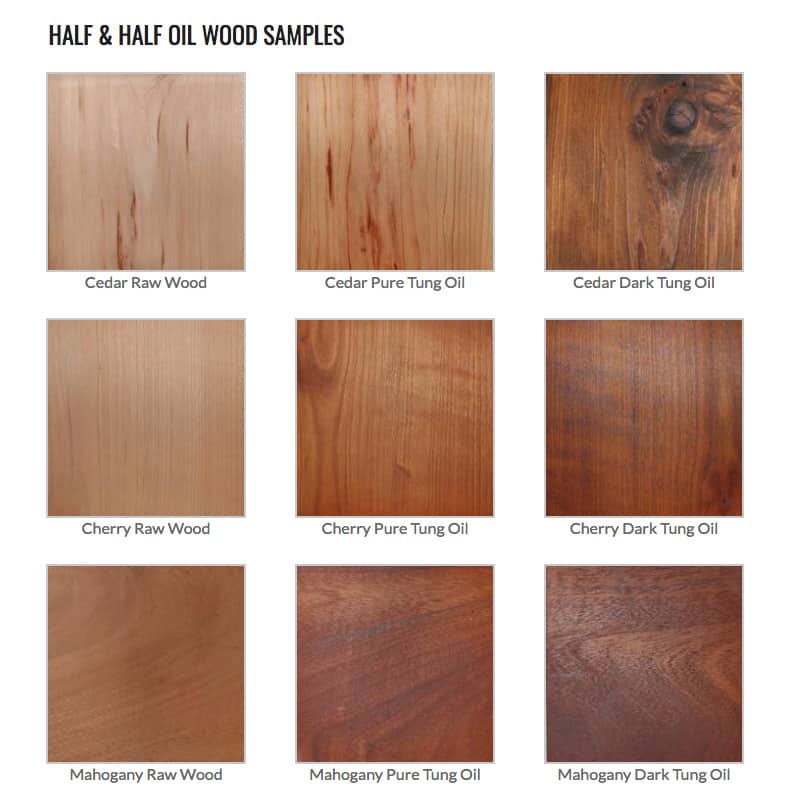This detailed close-up photograph showcases nine square images of wooden surfaces treated with varying levels of oil, arranged in a 3x3 grid under the title "Half and Half Oil Wood Samples" in black capital letters. Each row displays a different type of wood: Cedar, Cherry, and Mahogany, progressing from untreated raw wood on the left to lightly oiled in the middle, and heavily oiled on the right. 

From the top left, the images and their labels read as follows:
1. Cedar Raw Wood: A light-colored wood with minor darkening.
2. Cedar Pure Tongue Oil: The wood is slightly darker with more visible grain.
3. Cedar Dark Tongue Oil: The wood has a significantly darker, rich tone highlighting its natural deformities.

In the second row, the progression is visible for Cherry Wood:
1. Cherry Raw Wood: A light wood, similar to Cedar but with more pronounced grain.
2. Cherry Pure Tongue Oil: The wood takes on a dark reddish-orange tint, characteristic of cherry wood.
3. Cherry Dark Tongue Oil: The wood is even darker than the previous, with a deeper cherry color.

In the bottom row, the stages for Mahogany Wood are depicted:
1. Mahogany Raw Wood: A noticeably darker wood compared to Cedar and Cherry.
2. Mahogany Pure Tongue Oil: The wood is enriched with a very dark, rich oil.
3. Mahogany Dark Tongue Oil: The wood achieves a profound dark reddish hue, showcasing the deepest treatment stage.

The arrangement effectively contrasts the lightest raw woods to their darkest oiled counterparts, emphasizing the transformative impact of oil treatments on wood color and texture.